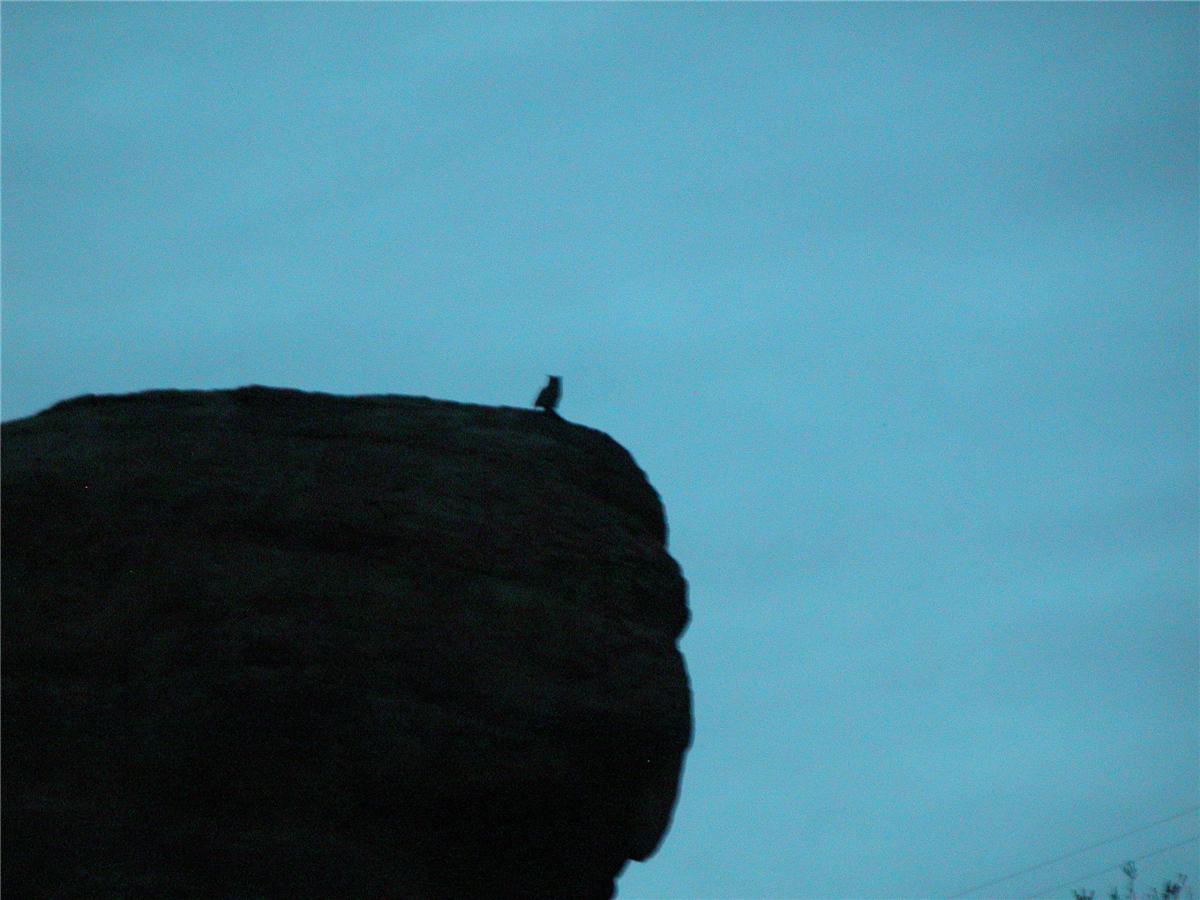This photograph captures a dramatic and natural scene featuring a rock formation and a silhouette of an owl set against a predominantly blue, slightly cloudy sky. The image is taken from below, providing a unique upward perspective on a cliff with uneven, layered edges that project outwards into the center of the photo. In the lower left-hand quarter of the image, the dark rock formation is prominent and extends roughly a fourth of the photograph. At the very edge of this formation perches an owl, whose silhouette stands out against the simple and unobstructed blue sky background. Despite the image's overall simplicity and somewhat blurred quality, additional details include faint traces of two power lines and the tips of a tree visible in the lower right-hand corner, lending a touch of the modern world to this otherwise natural and serene scene.